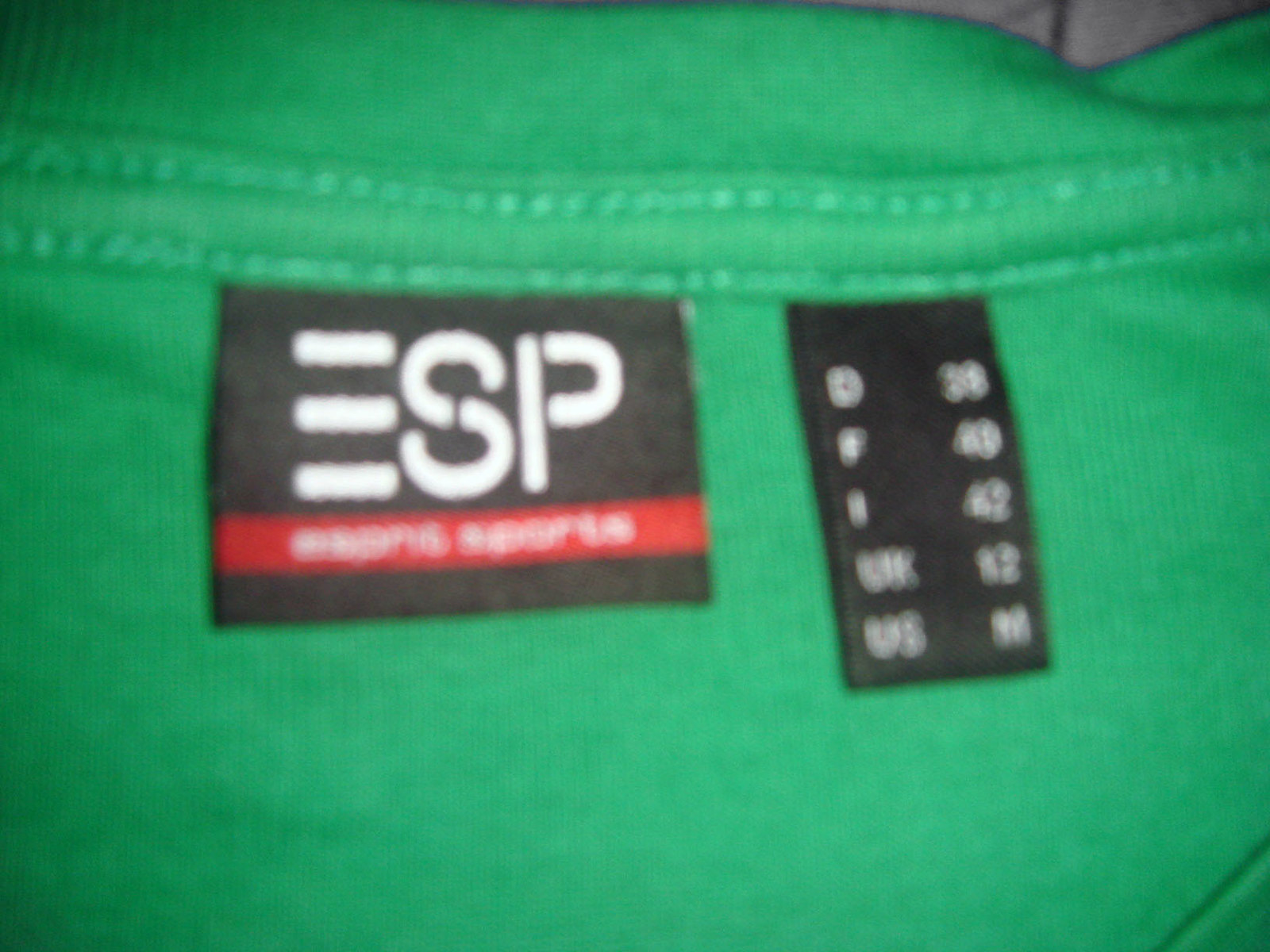The photograph displays a close-up shot of an emerald green garment, likely the inside of a shirt just below the collar, characterized by double lines of green stitching running horizontally across the top. At the upper edge of the image, there is a slight triangular fold showing a gray lining behind it. Prominently positioned is a black rectangular label with a company logo, "ESP," in stylized white letters, accompanied by a red stripe below it containing white text that partially reads "something sports," though the first word is indistinct due to blurriness. Adjacent to this label is another black tag displayed vertically, detailing the shirt’s sizes in various countries: for the UK, size 12; Italy, size 42; France, size 49; the Dominican Republic, size 38; and the US, size M (medium). The image is somewhat blurry, especially around the smaller text, but these key details are discernible.